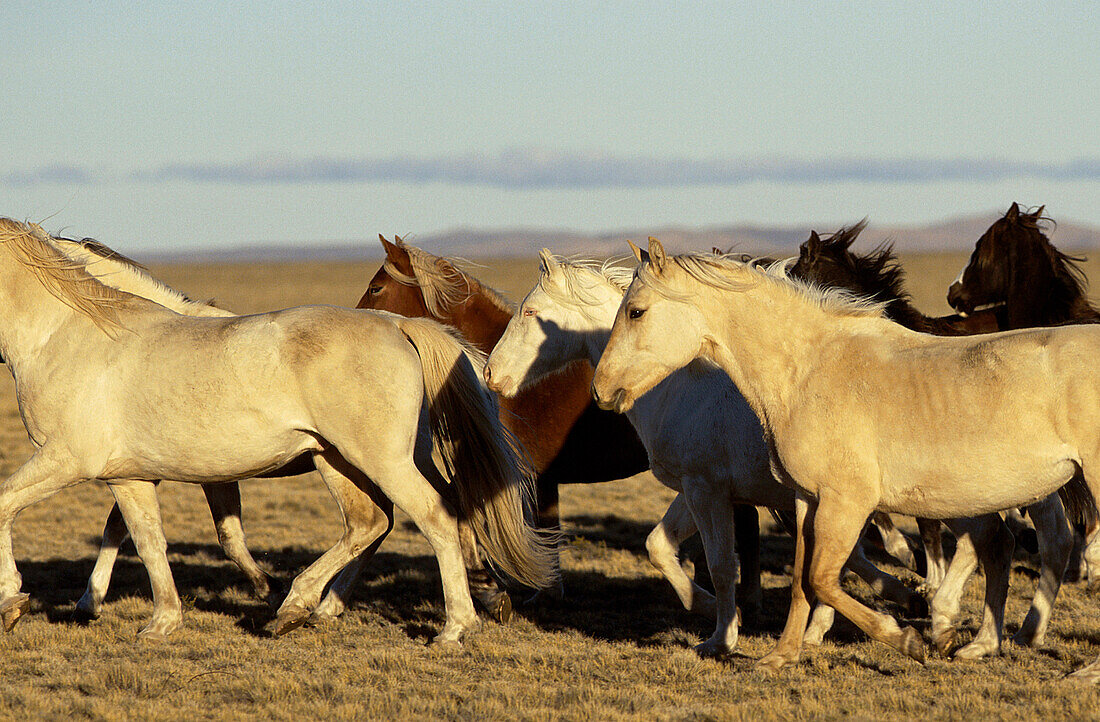This high-resolution photograph showcases a herd of seven wild horses trotting across a wide, open plain. The ground, covered in dry, loose grass that ranges from gold to brown, stretches across the lower half of the image. Above this, a thin line of mountains and wispy gray clouds cut across the sky, which is a pale blue. The horses mostly move in the same direction, towards the left of the image, with a few dark-colored ones oriented differently. The diverse herd includes a brown horse with a yellow mane, a white horse with a white mane, and a tan horse with an off-white mane among them. The foreground horses, some cream and beige, others dark brown, appear to be evenly sized, although their legs look slightly shorter, hinting they might be ponies. The serene yet dynamic scene captures the essence of untamed nature under a vast, open sky.